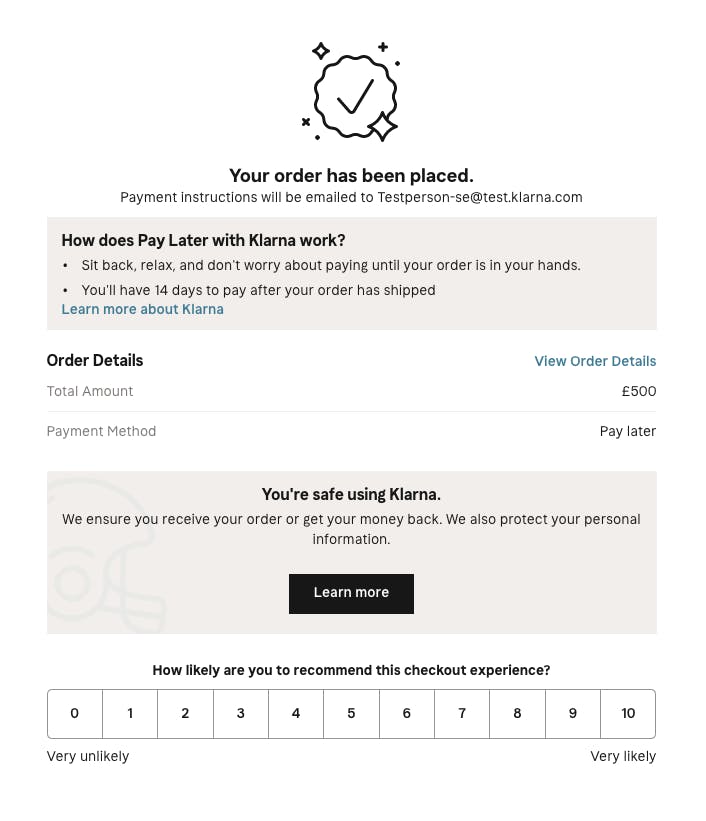The image starts with a distinctive icon at the top, featuring an irregular, wavy circle outlined in black with a white check mark in the center. Surrounding the icon are small boxes and plus signs. Below this icon, in bold black font, the text reads, "Your order has been placed." Underneath this, in regular black font, it states, "Payment instructions will be emailed to testperson-e at test.klarna.com." Both lines of text are centered beneath the icon.

Following this section, there is an off-white horizontal rectangular box. At the top left of this box, in bold black font, the heading reads, "How does Pay Later with Klarna work?" Here, "Pay," "Later," and "Klarna" are capitalized. The box continues with bullet-pointed, non-bold text detailing the service: "Sit back, relax, and don't worry about paying until your order is in your hands." and "You'll have 14 days to pay after your order has shipped." At the bottom of the box, in turquoise font, there is a clickable link: "Learn more about Klarna."

Below this, there is a white section with the heading "Order Details" in bold black font on the left. On the right side, in smaller turquoise font, it reads, "View order details." Under the "Order Details" heading, in light black font on the left, it states, "Total Amount." To the right of this, the cost is displayed as "£500." Further down, still on the left side, it says, "Payment Method," while on the right, in black font, it reads, "Pay Later."

Next, there is another off-white horizontal rectangular box, slightly wider than the first one. Centered at the top, in bold black font, it declares, "You're safe using Klarna." Beneath this, on the left side in non-bold black font, it ensures customers, "We ensure you receive your order or get your money back. We also protect your personal information." The word "information" is centered under "You're safe using Klarna." Below this text, there is a centered "Learn More" button with white font on a black background.

Finally, on a white background under this box, in bold black font, it asks, "How likely are you to recommend this checkout experience?" Below this question is a range from 0 to 10, each number in its own vertical rectangular box. Under the numbers 0 and 1, it reads "Very Unlikely," and under the numbers 9 and 10, it reads "Very Likely."